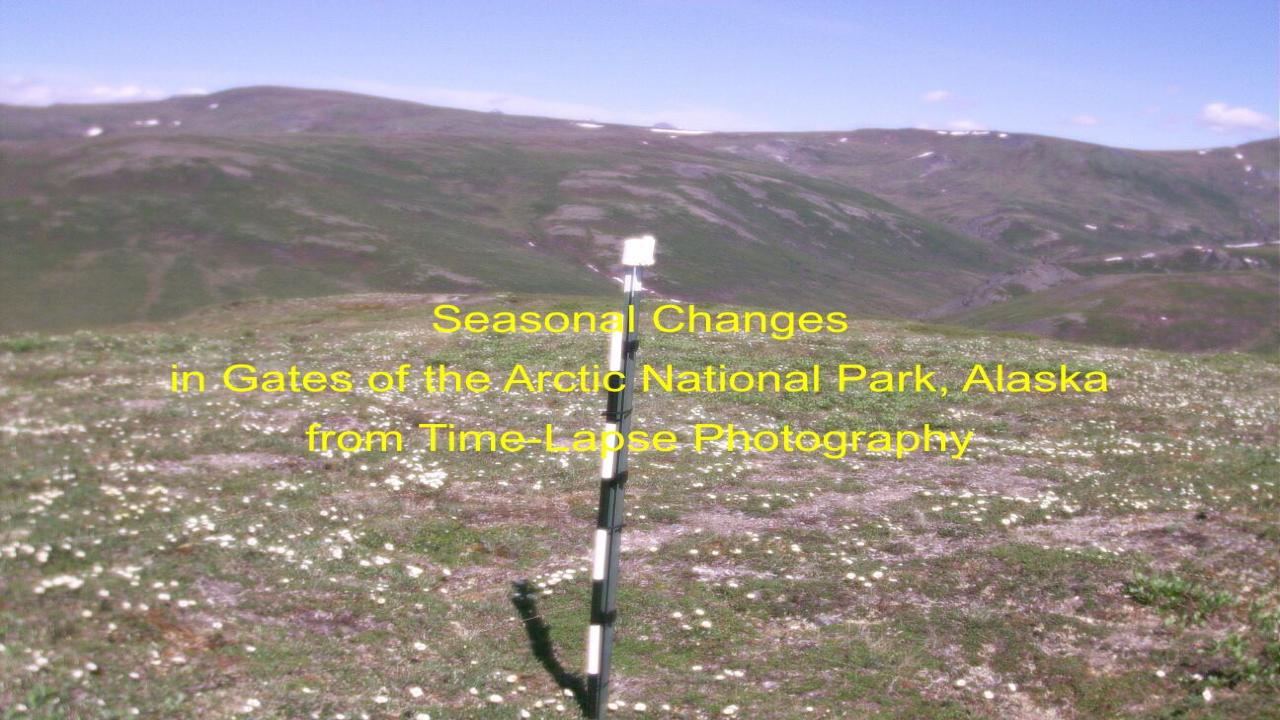The photograph captures a desolate yet stunning landscape in Gates of the Arctic National Park, Alaska, showcasing a tundra environment at the top of a mountain. The terrain is hilly and rocky, dotted with small white flowers and green lichen, with a mix of bare earth and sparse greenery. Central to the image is a fence post or vertical pipe, rising about two-thirds up the image, with one dark green section and another adjacent pipe that is black and white. The expansive scene also includes peaks and valleys in the distance, all under a bright blue sky with a few fluffy white clouds, suggesting it could be spring or summer. Overlaid text in yellow reads, "Seasonal changes in Gates of the Arctic National Park, Alaska from time-lapse photography," indicating the image might be a still from a time-lapse video. The photograph, though not high-definition, effectively conveys the raw beauty and isolation of the Alaskan tundra.